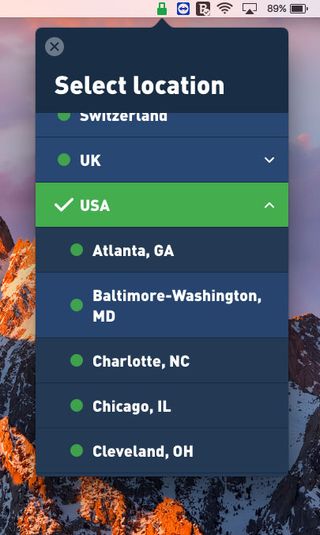Screenshot of a MacBook displaying a VPN application with a green highlighted lock symbol indicating secure connection. The app allows the selection of various locations, with an active VPN connection to the USA, denoted by a fully green checkmark. The drop-down menu under the USA option reveals several specific cities including Atlanta, Georgia; Baltimore, Maryland; Charlotte, North Carolina; Chicago, Illinois; and Cleveland, Ohio. Additional selectable locations like Switzerland and the UK are marked with green dots. In the background, a picturesque scene of a purple sky and a snowy brown mountain is visible. The MacBook shows an 89% battery level, active WiFi connection, and a screen-sharing option, with all text displayed in white.